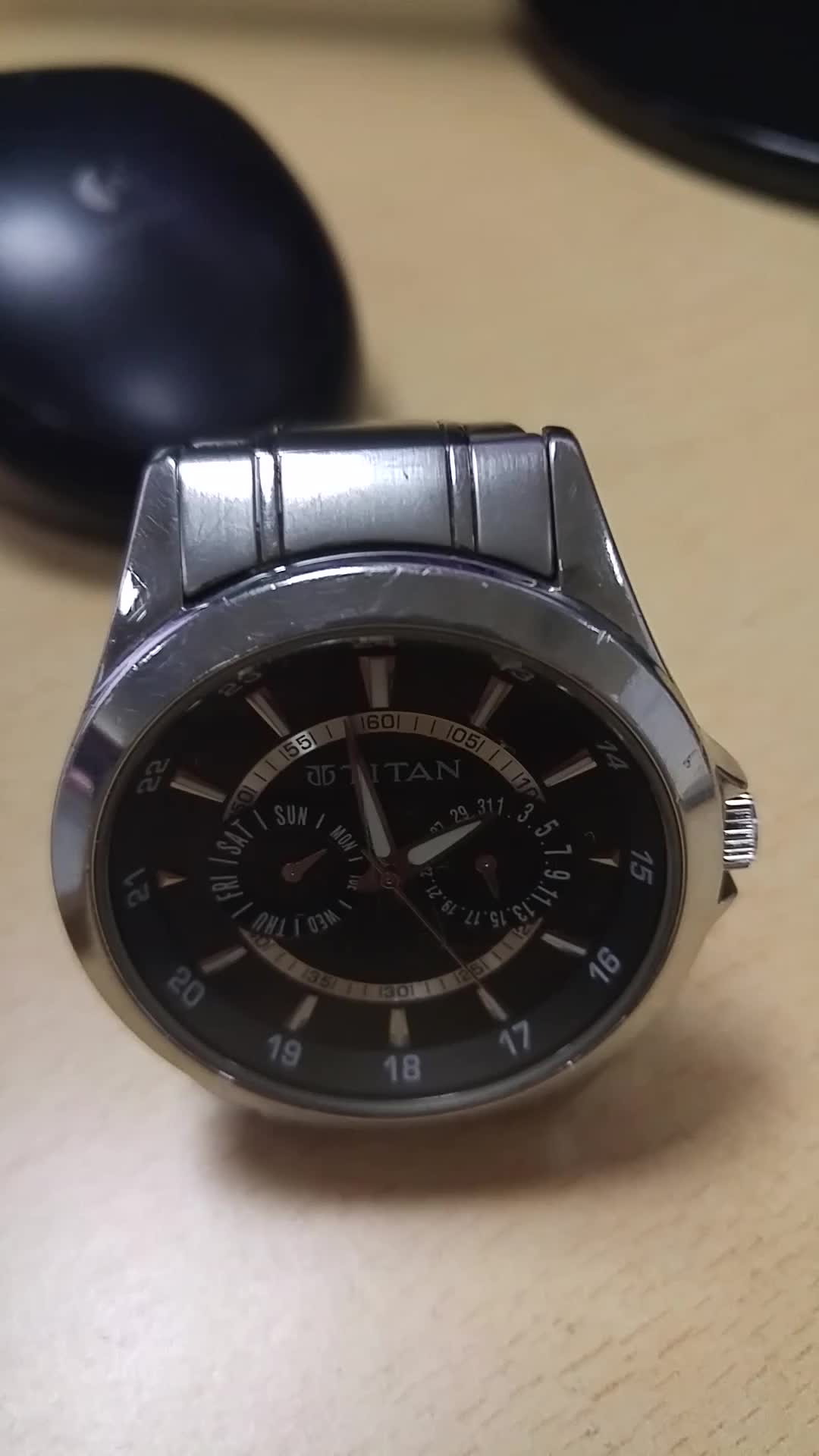An overhead, close-up image depicts a well-worn, stainless steel wristwatch standing upright on its side against a hard, cream-colored surface. The watch's metallic band is slightly visible at the top. The black watch face, encased in a silver, somewhat scratched bezel, features an intricate design with multiple inlaid dials. The main face includes gold hour markers and a smaller, reflective inner dial with markings from 1 to 60 for the seconds. The watch has pointed triangular hands and a second hand that is slender and red. Above the hands, the brand name "Titan" is visible. To the right of the watch face, there's a winding crown. In the background, a black computer mouse with a gray button is partially visible in the top left corner of the image, and a small black circle—possibly a stand—is seen entering the frame from the top right.